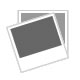The image depicts an elaborate album cover designed for a three-disc holiday music collection. The cover features a visually engaging background that transitions from white near the top to gray on the sides, with partial imagery of a pomegranate and some grapes layered with green spots. The top of the cover includes an image of a book and three lifesaver-like objects in a box, setting a festive tone. Prominently written in red at the top are the titles "Cocktail Crooners" and "Entertaining Holiday Fare," surrounded by meticulously listed holiday tracks.

The album includes a wide array of classic Christmas songs, detailed in a neat, numerical listing with song titles in green and artist names in red. Tracks featured include "The 12 Days of Christmas" by Bing Crosby and The Andrews Sisters, "Oh Come All Ye Faithful" by Perry Como, "Here Comes Santa Claus" by Bing Crosby and The Andrews Sisters, "Jingle Bell" by Glenn Miller, and many more. Each disc in the collection is illustrated and described, emphasizing the album's festive and elegant nature.

The back cover contains text extolling the collection as the ultimate holiday party accompaniment, complete with tips and recipes, ensuring a celebration filled with cheer. The vivid, colorful design of the cover, accented with green, brown, and cream hues, and the detailing of the track listings highlight the album's dedication to bringing festive joy and nostalgia through its music.